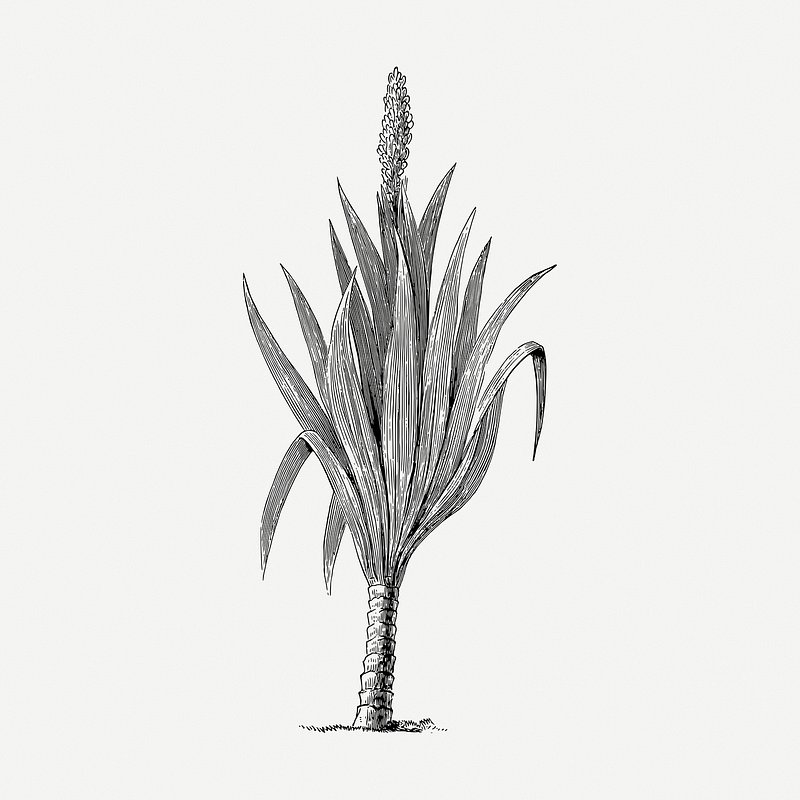The image depicts a detailed, hand-drawn ink sketch of a plant with a rigid, palm tree-like stem that is marked by circular rings. The stem, firm and straight, rises a few inches from the ground before it gives way to a cluster of long, slender leaves. These lengthy leaves, reminiscent of traditional weed leaves, arch and bunch together, creating a dense foliage. At the apex of the plant, a single tall, spiky flower blooms, though its specific type and color are indiscernible due to the monochrome palette. The entire drawing is rendered in shades of gray and black, set against a plain, light gray gradient background, lending a timeless quality to the illustration. The centralized position of the plant commands focus, with no additional elements or text present to distract from its intricate details.